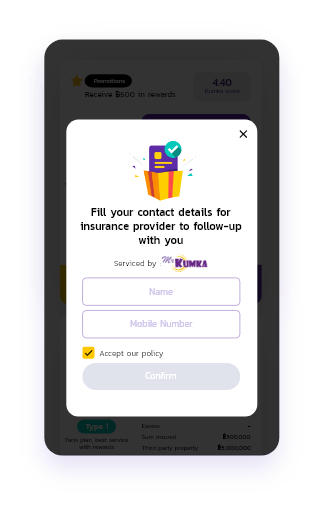The image features a gray background with a prominent gold star in the upper section, highlighted with a 4.40 rating. Below the star, text reads "Receive $5 Rewards." A white window in the center of the composition contains the word "PURPLE" in bold letters. Adjacent to this text is a green checkmark symbol, signifying completion or approval.

Additionally, there is a message box with a title labeled "Fill Your Contact Details for Insurance Provider to Follow Up with You." This section is serviced by a company named "Gunka." The form fields include a space for the name, denoted as [Name], and a mobile number, indicated as [Mobile Number].

Further down, there is a yellow checkbox that reads, "Accept Our Policy," which users are required to tick. It appears to be next to a placeholder section for a friend's reference, labeled "Physical Friend" with an example entry starting with the letter 'J.'

The image also includes a financial section indicating coverage details: "$300,000 Third-Party Property" and "$1,000,000 Coverage." The overall layout is punctuated with professional and organized elements, geared towards facilitating insurance policy acceptance and registration.